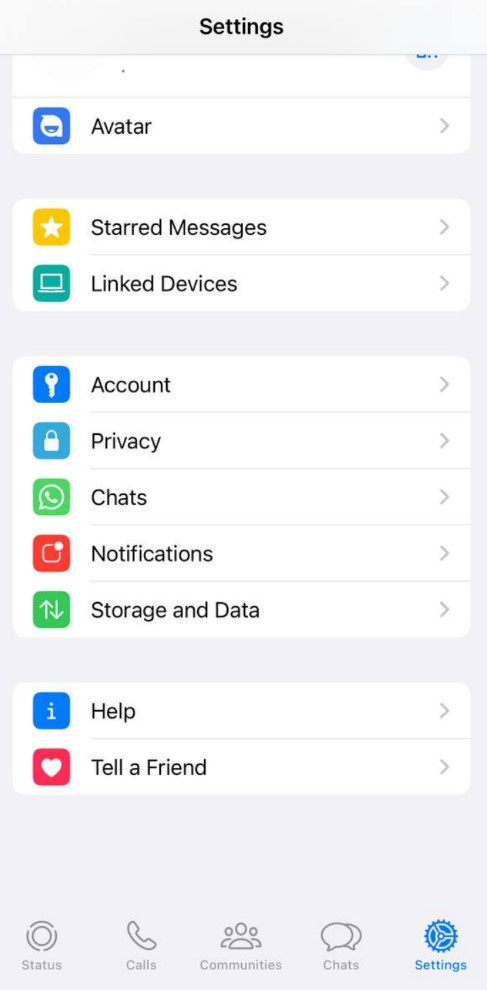This is a detailed and cleaned-up caption for the described image:

The image is a cell phone screenshot featuring the 'Settings' menu of an application. The screenshot has a gray background, with the top section in black displaying the word "Settings" in white. Below this, there is a list of menu items in black text on a white background, each accompanied by an arrow icon on the right.

The items listed in the menu, from top to bottom, are:
1. **Avatar** - Icon: A mouth
2. **Starred Messages** - Icon: A yellow star
3. **Link Devices** - Icon: A computer
4. **Account** - Icon: A key
5. **Privacy** - Icon: A padlock
6. **Chats** - Icon: A messaging bubble (WhatsApp message icon)
7. **Notifications** - Icon: A square with a circle
8. **Storage and Data** - Icon: An up and down arrow
9. **Help** - Icon: A white letter "I"
10. **Tell a Friend** - Icon: A heart

At the bottom of the screen, there is a gray navigation bar with tabs labeled "Status," "Calls," "Communities," and "Chats," all in gray, while "Settings" is highlighted in blue.